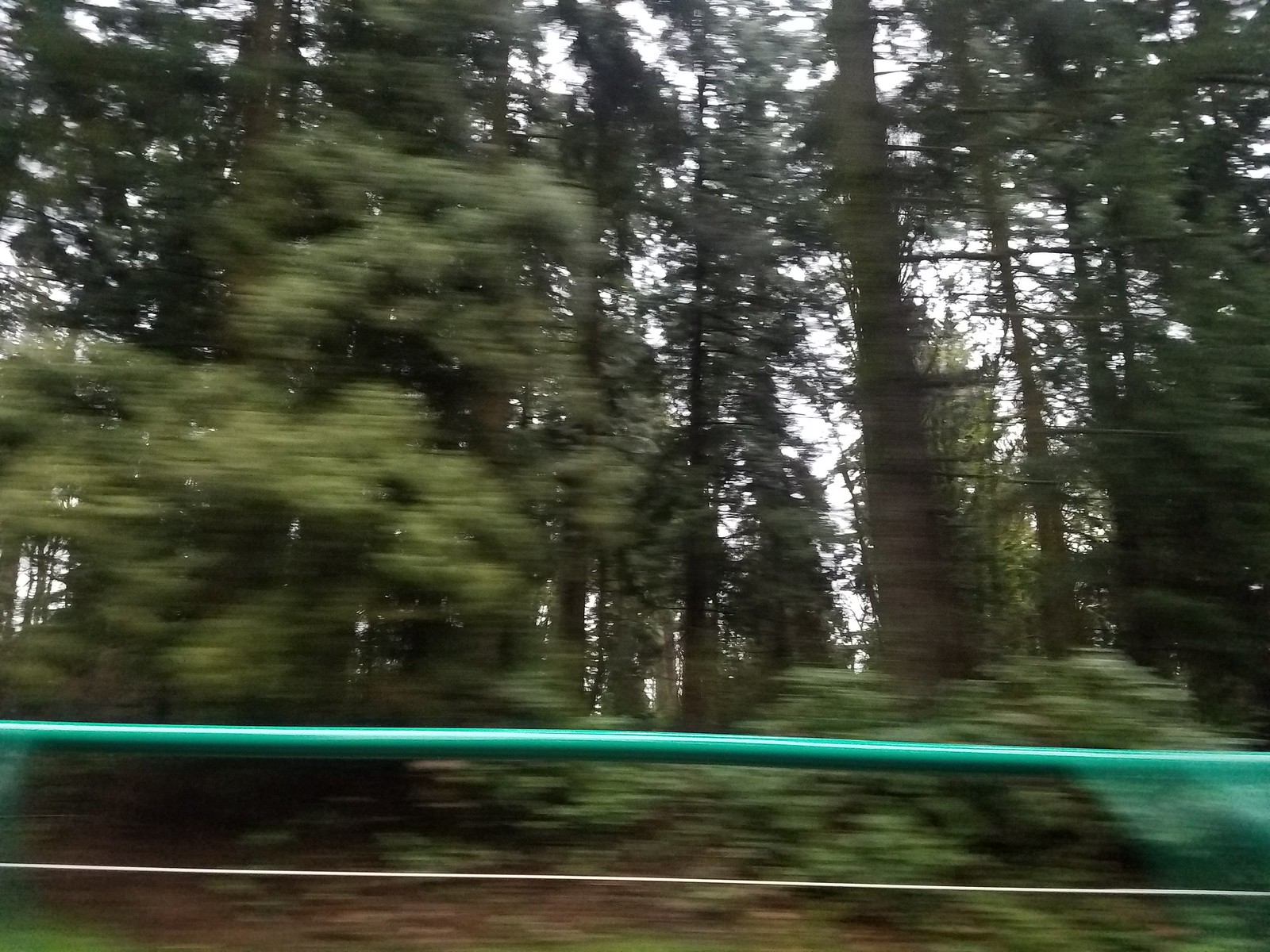This is a square color photograph of a forest captured in motion, likely from a moving vehicle. The image is predominantly blurry, but some parts of the trees are slightly more in focus. The upper five-sixths of the photograph showcase tall, mainly dark green trees with brown trunks, some of which have broader shapes and lighter-colored leaves. The background features a mix of backlit and more vividly green trees, set against a hazy gray sky. 

In the lower part of the image, there is a distinct green horizontal line running from left to right, about a third from the bottom. This line has a metallic sheen, suggesting it might be part of a barrier seen through a vehicle window. Below this, parallel and closer to the edge, is a thin white line that could be a drawn artifact or possibly a thin rope. The ground beneath the trees is a patchwork of dark brown earth and green underbrush, contrasting with a strip of bare brown earth running along the bottom of the photograph.